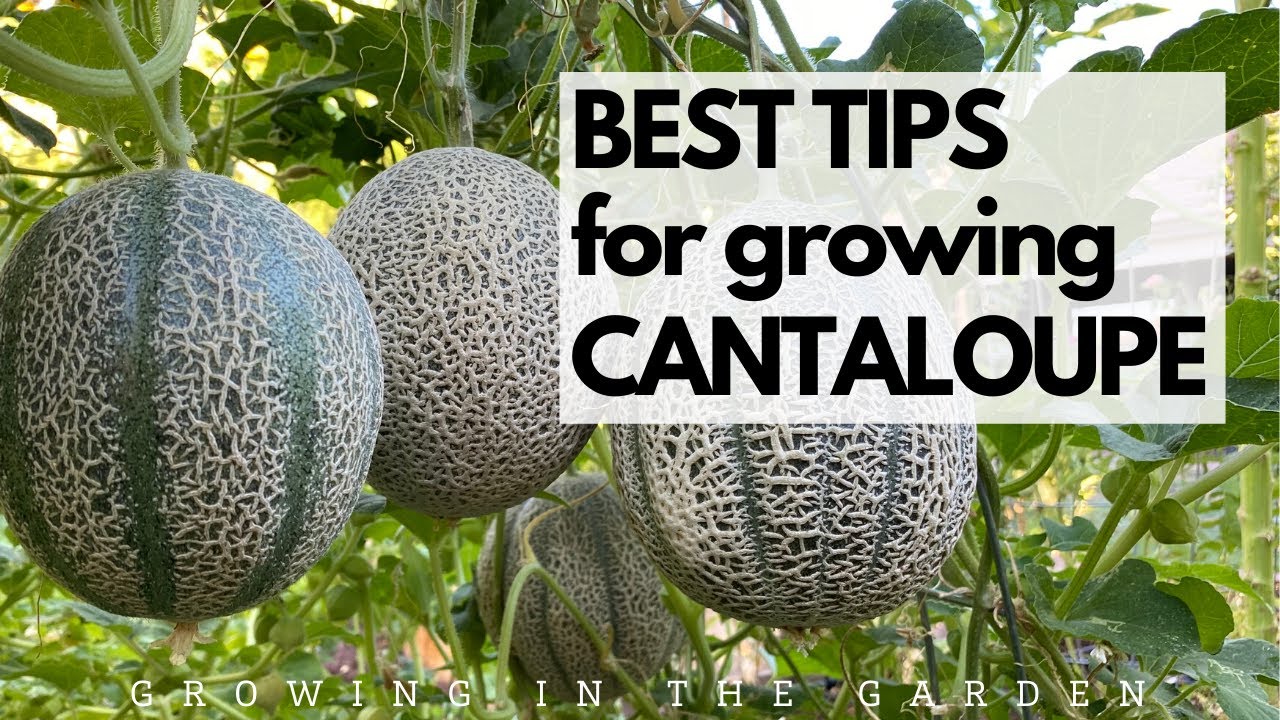The horizontally rectangular image showcases three cantaloupes hanging from vines amidst dense foliage with slices of the sky peeking through in the upper right corner. In the foreground are the cantaloupes: the one on the left displays a typical beige netted skin with distinct vertical green stripes, similar to a basketball; the middle cantaloupe features a standard cantaloupe appearance without any stripes; and the one on the right has lighter, less pronounced green stripes. At the bottom border, the text reads "Growing in the Garden," while a large white box with black writing in the center states "Best Tips for Growing Cantaloupe." The image is likely a cover for a book or an article on gardening.